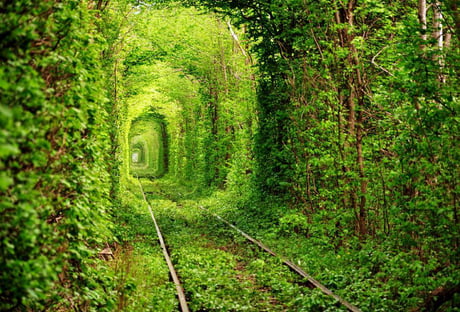This image is a captivating outdoor photograph of an abandoned railroad track that vanishes into an overgrown, verdant tunnel. The scene is dominated by a lush canopy formed by smaller deciduous trees, their green leaves arching overhead to create an almost oblong, tunnel-like effect. In the foreground, the two clear railroad tracks run straight into the heart of this green corridor, flanked by slender brown tree trunks and dense foliage on either side. The right side of the tracks displays a detailed view of darker green leaves, while the left side presents a softer, more out-of-focus expanse of greenery. Brown earth and sprouting grass cover the ground adjacent to the tracks. Light filters through the leafy archway, casting a spectrum of light and dark greens with occasional patches of yellow. Sunlight peeks through the canopy, illuminating parts of the tunnel and creating a striking optical illusion. The overall scene emits a primordial ambiance, suggesting a place once traversed by trains, now reclaimed by nature.